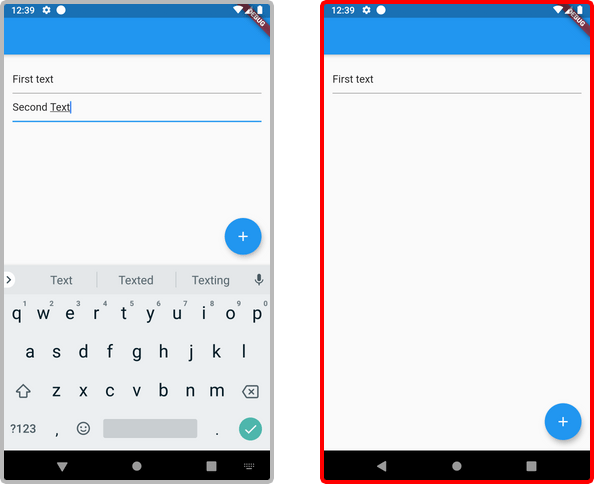This image comprises two mobile phone screenshots, both displaying what appears to be the same webpage, though with slight variations. 

In the left screenshot, the webpage has a blue header at the top-left corner featuring the number "1239". Beneath this header, the page is primarily a white background. There are two lines of text: "first text" and "second text". The cursor is positioned just after the "T" in "second text," which is underlined in blue. Below the text area, there is a QWERTY keyboard. Above the keyboard, there are word suggestions: "text," "texted," and "texting," flanked by a microphone icon on the left and an add/plus button on the right. 

The right screenshot, outlined in red, follows a similar format with a blue header and a white background. This version has less text, showing only the line "first text" in black. At the bottom-right corner of the screen, there is a blue button with a plus sign inside it. The remaining space appears to be blank.

Both screenshots depict different states of the same webpage interface focusing on text input functionality.